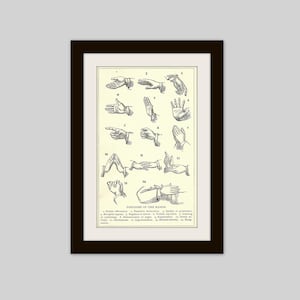The image is a black and white sketched illustration framed in a black wooden frame with a white matting. It depicts various hand signs, possibly sign language or different hand gestures, including a handshake, pointing finger, prayer hands, open palm, and high five, among others. The illustration features about 14-15 different hand positions, each marked with a letter or number next to them. Though the text at the bottom explaining the gestures is blurry and illegible, it indicates that each hand sign has a specific meaning or context. The background of the image appears to be a cream color, and the detail is meticulously outlined in black, giving it a clean, instructive appearance. The frame is set against a white or eggshell-colored background, making the illustration stand out prominently.